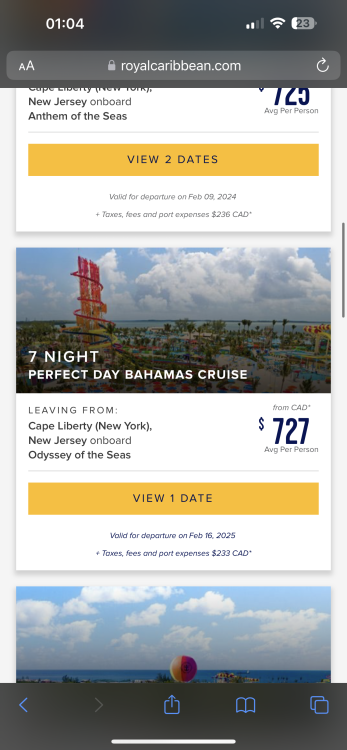A smartphone screen displays a webpage from royalcaribbean.com. The device indicates a 23% battery level and the time is 1:04 PM. At the top of the screen, a gray URL bar reveals the web address. The webpage shows various vacation packages offered by Royal Caribbean. The first listing is partially visible, showing "New Jersey on board, Anthem of the Seas," with additional details cut off. Below it, an orange bar states "view two dates." The next visible listing is a "Seven Night Perfect Day Bahamas Cruise," featuring an image of a cruise ship with visible waterslides, the sea, and clouds in the background. The text notes the price as $727 per person, departing from Cape Liberty, New Jersey, onboard the Odyssey of the Seas. The final image shows parts of a cruise ship with a red and yellow bubble, the ocean, and a blue sky with white clouds. The bottom of the screen has a black bar with various blue icons outlined in white.